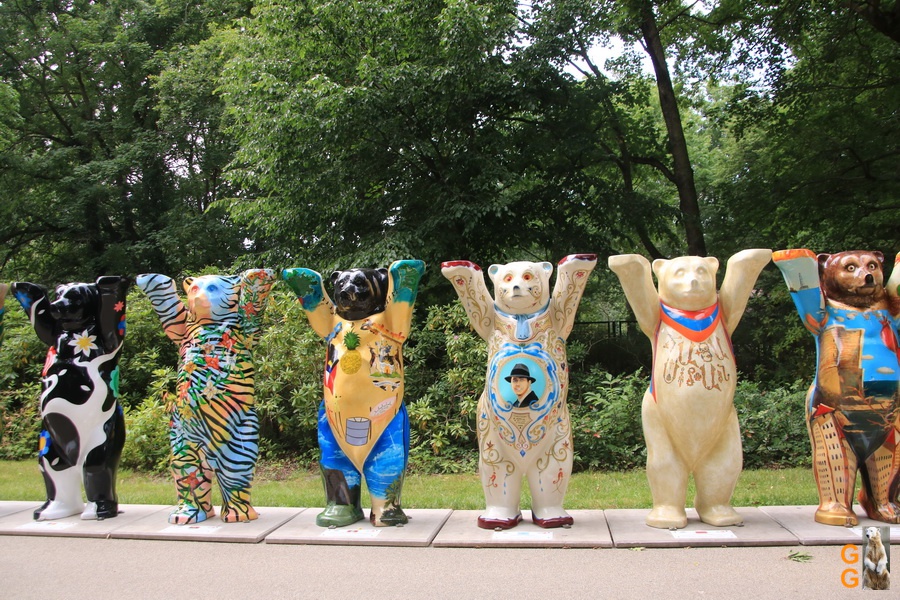The image depicts a row of six life-sized bear statues, positioned on a sidewalk with their arms raised towards the sky. These bears, standing on hind feet, are all uniquely painted and exhibit a variety of colors and designs. From left to right, the first bear is black with white spots and features small flower details. The second bear resembles a blue tiger with orange accents. The third bear is creatively styled in a yellow shirt, blue pants, and boots, resembling Woody from Toy Story, with a black head and green paws. The fourth bear is white with a detailed image of a man wearing a hat on its belly. The fifth bear is cream-colored, and though it has some unreadable lettering, it features visible designs. The sixth bear is brown and appears to be wearing a blue shirt and patterned pants. Surrounding this vibrant display are large trees with dark green leaves, suggesting a nearby forest, and some lower shrubs, providing a natural backdrop.